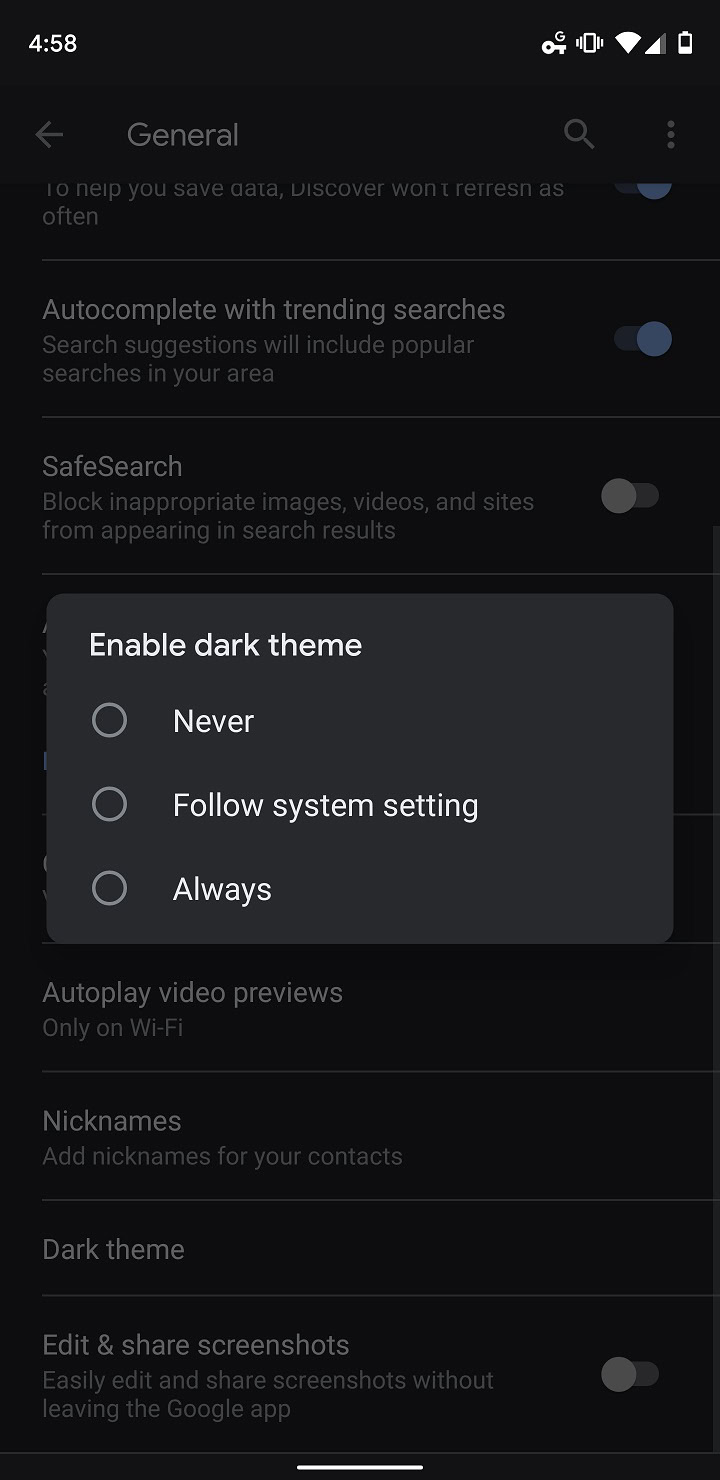This detailed caption describes a screenshot from a settings application, providing an in-depth look at the image:

The screenshot is taken from a settings application, with the title "General" prominently displayed at the top. The current time shown on the device is 4:58. On the left side of the header, there is a back button, and on the right side, there are search and menu icons, the latter represented by three vertical dots in a line. The settings interface contains various sections:

1. **Auto-complete with Trending Searches:** This feature is enabled, as indicated by the active toggle switch. The description beneath reads, "Search suggestions will include popular searches in your area."

2. **Safe Search:** This option is designed to block inappropriate images, videos, and sites from appearing in search results. However, the toggle for this function is turned off.

In the middle of the screen, a pop-up window is prominently visible, prompting the user to "Enable Dark Theme." The pop-up offers three selectable options: 
- Never,
- Following system setting,
- Always.

Below the pop-up, additional settings options are visible but not currently active:
- **Autoplay Video Previews,**
- **Nicknames,**
- **Dark Theme (presumably a duplicate setting outside the pop-up),**
- **Edit and Share Screenshots,** the latter of which is turned off.

This comprehensive description captures the structure and content of the settings application screenshot in detail.